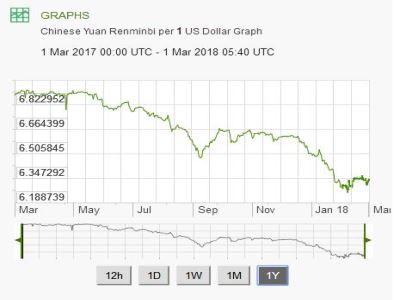The image showcases a detailed graph titled "Graphs" in thin, wide, green capital letters positioned in the upper left corner. Adjacent to this text, there is a small icon depicting a graph over a grid. Below, in gray text, it specifies, "Chinese Yuan Renminbi per one U.S. dollar graph," and provides a time frame from "1 March 2017, 00:00 UTC to 1 March 2018, 05:40 UTC."

The graph displays vertical numerical markers on the y-axis at intervals: 6.188739, 6.347292, 6.505845, 6.664399, with the highest point marked at 6.822952. The horizontal axis (x-axis) is labeled with months: March, May, July, September, November, and January 18th.

The plot of the price fluctuations is represented by a dark green line against a light gray grid background. Below this main graph, there is a compressed version of the same graph, distilling the data into a shorter, vertically compact format. This condensed graph is unlabeled but includes a selection option at the bottom, highlighting "12 hours, one day, one week, one month," with "one year" being selected.

Additionally, this lower graph features green bars with arrows on either end, allowing users to toggle between different time frames or data views.